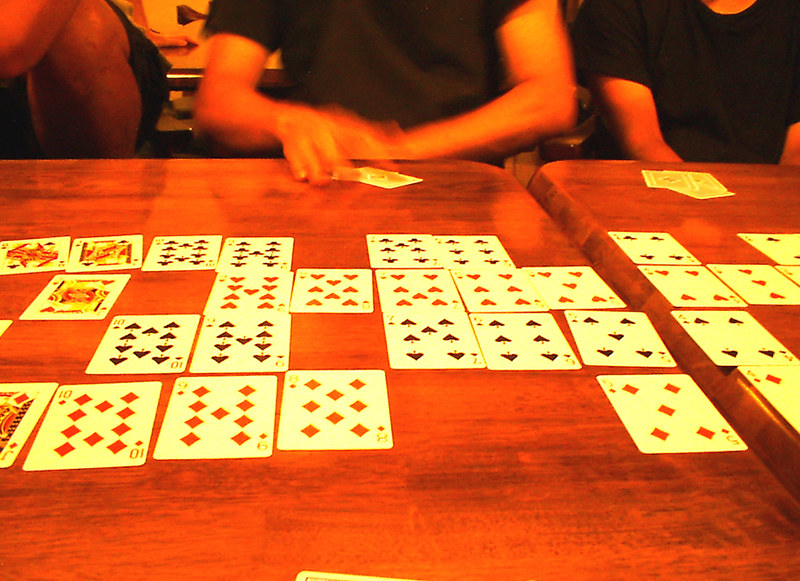A vivid, close-up photograph captures the intense moment of a card game in progress. The scene unfolds on what appears to be two tables pushed together, the composite table bathed in a reddish hue that might be a trick of the lighting, as it could actually be brown. In the foreground, playing cards are meticulously arranged face-up in a pattern, predominantly showcasing number cards, with a few Jacks and Kings interspersed. The cards are both red and black, creating a striking visual contrast.

To the right of the image, two individuals are engaged in the game, both clad in short, black-sleeved shirts. The person across the table from the photographer is clearly visible, mid-action, placing a card onto the table. The second player has their hands obscured beneath the table but has several cards directly in front of them. A hint of a third person is visible in the far left corner, though their features are indistinct. The overall composition of the photograph, combined with the dramatic lighting, conveys a sense of concentrated engagement and a fervent atmosphere.